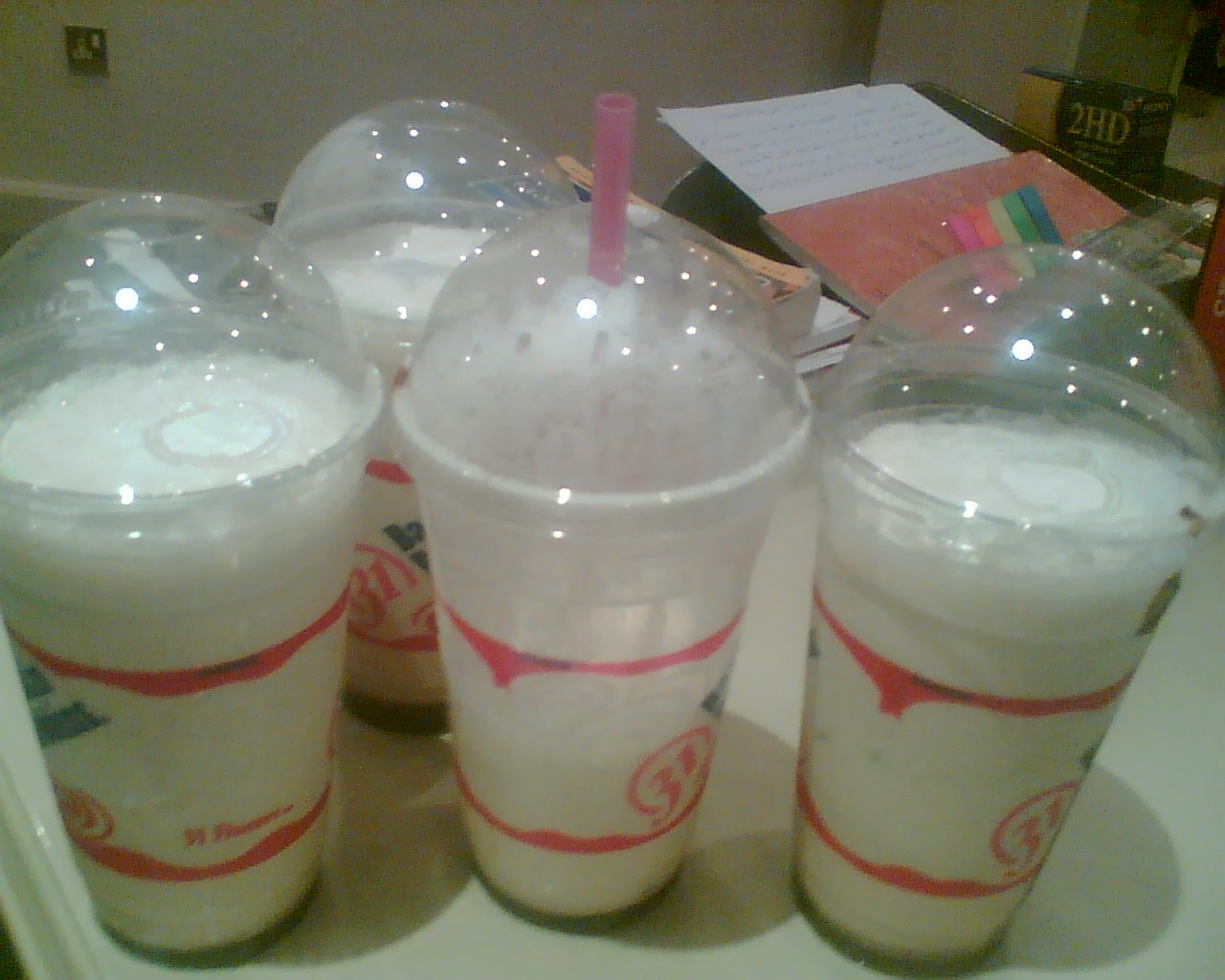This close-up photograph captures four transparent plastic milkshake cups, each adorned with a red "31" inside a circle and a dome-covered lid with a hole in the middle, indicative of Baskin-Robbins. They are set on a white surface, which could be the top of a small refrigerator or table. Three of the cups are completely filled with a white, vanilla milkshake-like substance, while the center cup contains a pink straw and is noticeably drained, with only about a third of its contents remaining. The bottom of each cup shows a faint greenish line of liquid. In the background, there are various objects that suggest a student's room, including papers, notebooks, highlighters, colorful crayons, study books, and a black box with gold accents bearing the label "2HD."